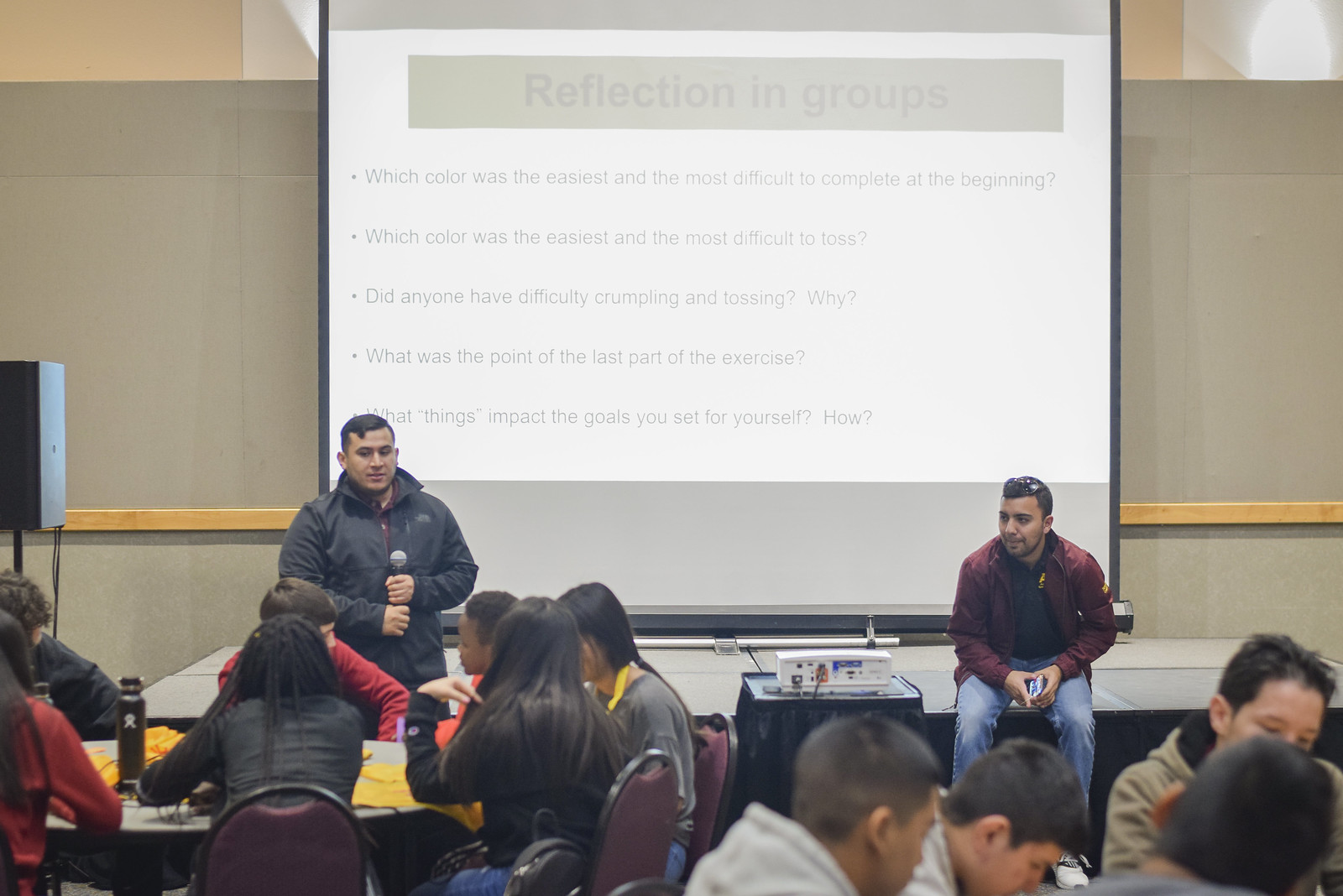The image captures a dynamic classroom or conference session centered around group reflection activities. Dominating the scene is a large projector screen, which spans from the top to nearly the entire height of the image. The screen displays a title page titled "Reflection in Groups," followed by a series of bullet-pointed questions: "Which color was the easiest and most difficult to complete at the beginning?", "Which color was the easiest and most difficult to toss?", "Did anyone have difficulty crumpling and tossing? Why?", "What was the point of the last part of the exercise?", and "What things impact the goals you set for yourself, how, or why?"

In the middle foreground, a man stands to the left holding a wireless microphone in his left hand. He wears a black jacket and has dark black hair. Facing him and seated on an elevated stage is another man with dark hair, clad in a maroon jacket and light blue jeans, who is slightly hunched over and also looking at the audience.

The room features several round tables populated by young men and women engaged in the session. The tables are surrounded by maroon and black chairs. The detailed setting and the interaction between the speakers and participants create a focused and engaged atmosphere.